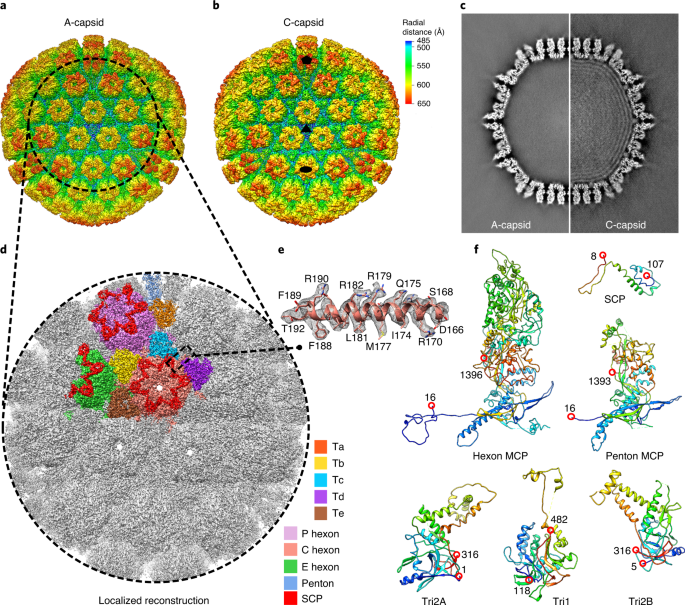The image is a detailed scientific diagram with multiple panels and intricate annotations resembling a cellular or viral structure represented in various colors and patterns. The upper part features two prominent, circular sections labeled "A capsid" and "C capsid", each showcasing rich, floral-inspired designs. Black dotted lines, marked with "localized reconstruction", link these sections to a lower area filled with numerous colored squares, each square marked with labels such as TA, TB, TC, TD, and TE. These squares are filled with various hues like orange, yellow, blue, purple, and brown. Additionally, there are labels such as hexon, penton, and different numbers like 1078, 1393 along with terms like pentonMCP, try2B, try1, 482, and P-hexon scattered throughout the image. The top right corner displays a grayscale section with thread-like textures, suggesting some form of structural analysis, possibly resembling an x-ray or detailed stitching. The complexity and variety of labeled elements such as colored splotches, numbers, and anatomical references indicate the image is a comprehensive reconstruction or visualization of a capsid topology, possibly aimed at scientific analysis of viral structures.